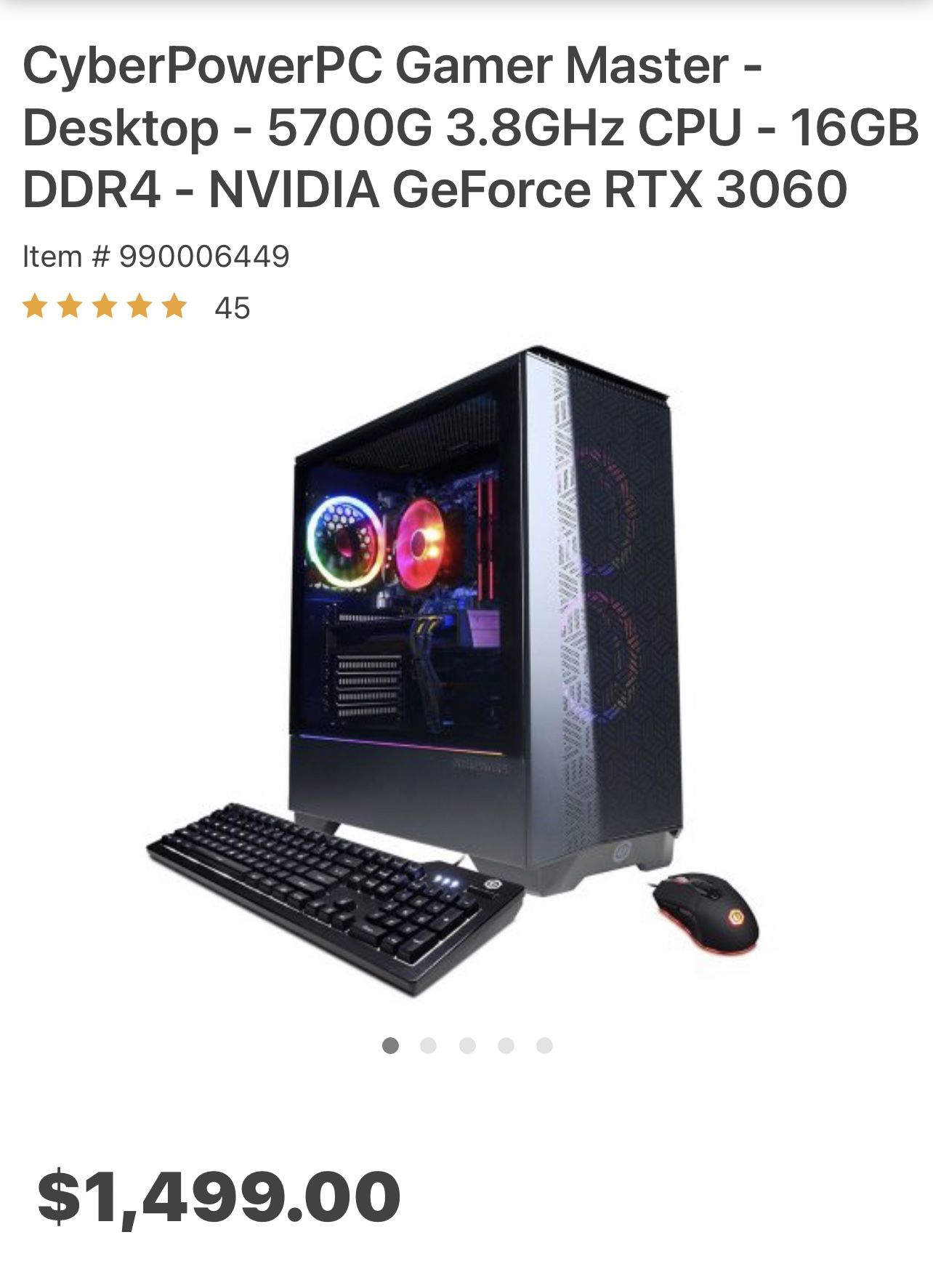This screenshot showcases part of a product page on a website featuring the "CyberPowerPC Gamer Master." At the top of the listing, the product title is prominently displayed, followed by key specifications: "Desktop, 5700G, 3.8 GHz CPU - 16 GB DDR4, NVIDIA GeForce RTX 3060." The item number is listed below these details. 

The product boasts a 5-star rating from 45 reviews, indicating high customer satisfaction. Further down, the page presents an image of the PC tower, which features colorful RGB fans and a sleek black case with a shiny, mesh-like front panel. Accompanying the tower is a black keyboard positioned alongside the side panel and a black mouse placed in front. The entire package is priced below $1499.